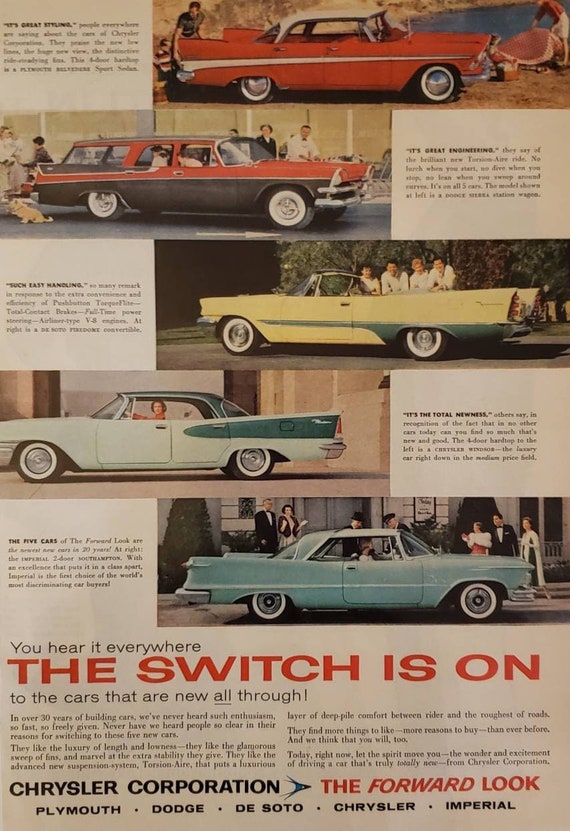This vintage magazine advertisement for the Chrysler Corporation showcases a vertical portrait-style layout with a series of images and accompanying text blocks showcasing the sleek, fin-tailed cars of the late 1950s to early 1960s. The page, though old and faded, is in great shape and filled with extensive text that may be challenging to read due to its small size. 

The top image features a red convertible with a white top, displayed at a lakeside picnic. Below it is a funky black and red station wagon set in a town street scene. The third car is a yellow convertible with a green stripe and the top down, captured in a lively setting. The fourth vehicle is a light blue, hardtop coupe with a dark green stripe, seen in a street scene. The final car at the bottom is a traditional 1950s sky blue sedan, situated at a formal event with people in tuxedos and gowns nearby.

Headlined in red, the advertisement reads, "You hear it everywhere. The switch is on." This vibrant catchphrase is followed by, "To the cars that are new all through," emphasizing Chrysler Corporation's innovative designs. At the bottom, it proudly mentions the brands under the Chrysler umbrella: Plymouth, Dodge, DeSoto, Chrysler, and Imperial, along with the tagline, "The Forward Look," highlighting the company's commitment to forward-thinking automotive design.